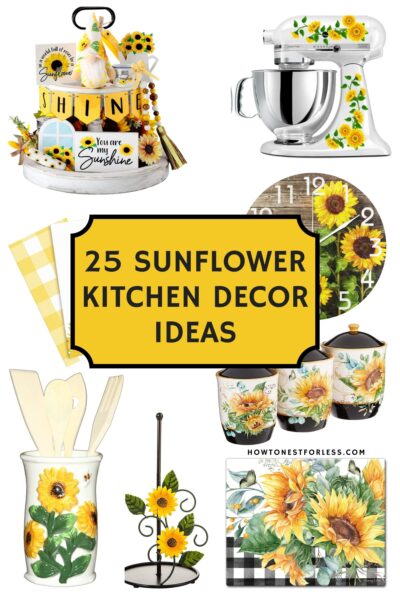This vibrant and detailed image showcases an array of sunflower-themed kitchen decor items, emphasizing a cheerful and rustic aesthetic. At the center, a yellow text box bordered in black, resembling a movie ticket, prominently displays the title "25 Sunflower Kitchen Decor Ideas." Surrounding this focal point, a variety of items are meticulously arranged. 

In the upper section, there's a traditional wooden clock with white hands, adorned with a sunflower design. Below it, a set of three canisters, varying in size, each featuring a sunflower print with black lids, hint at possible uses for storing sugar, spices, or tea. To the left, a white painted vase, decorated with sunflowers, holds an assortment of wooden kitchen utensils.

On the right side, a striking centerpiece is displayed on a white two-tier rack, including a yellow gnome with a "shine" sign and an array of sunflower-themed decor items. Adjacent to this is a sleek KitchenAid stand mixer, embellished with vibrant sunflower petals and green leaves. In the bottom right corner, a black and white checkered platter features a painted sunflower, while a wrought iron paper towel holder with a sunflower design stands nearby.

The overall color palette of the image is dominated by shades of yellow, black, and green, creating a cohesive and inviting atmosphere. The website name "howtonestforless.com" is subtly included below the items, suggesting a source for additional ideas. Overall, this image not only highlights specific sunflower decor items but also inspires a harmonious and sunny kitchen theme.